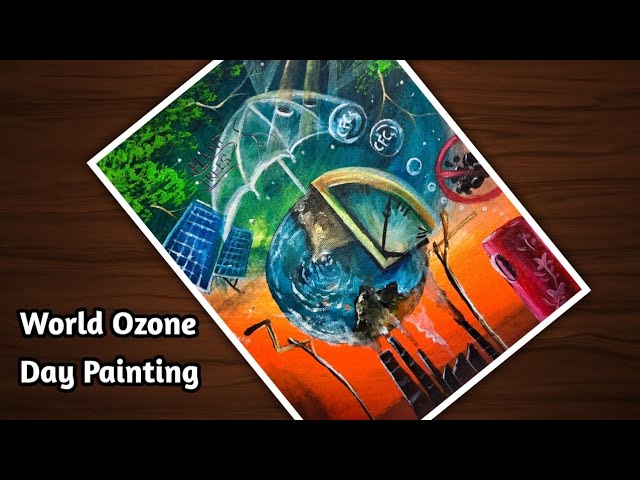The image, resembling a screenshot from a video with black bars on the top and bottom, features a vibrant and detailed painting tilted approximately 10-15 degrees to the left. Titled "World Ozone Day Painting" in white text on the left side, the artwork showcases a striking composition of various elements emphasizing an environmental theme. At the forefront is a large, clear umbrella with eyes on it, serving as a shield over a human figure, hinting at protection from environmental hazards. The background includes a vivid blue sky transitioning to an orange hue at the bottom, with a scattering of colorful bubbles containing letters. Prominently displayed are dark green rainforests, solar panels, and a dystopian landscape featuring dark buildings with smokestacks emitting black smoke. Additional details include a countdown clock on the earth, a can labeled with "CFC" inside bubbles, a prohibition sign over coal, and an encouraging message to "plant trees" with accompanying tree illustrations. The overall effect is a visually arresting, AI-stylized portrayal of the urgent need for environmental conservation.